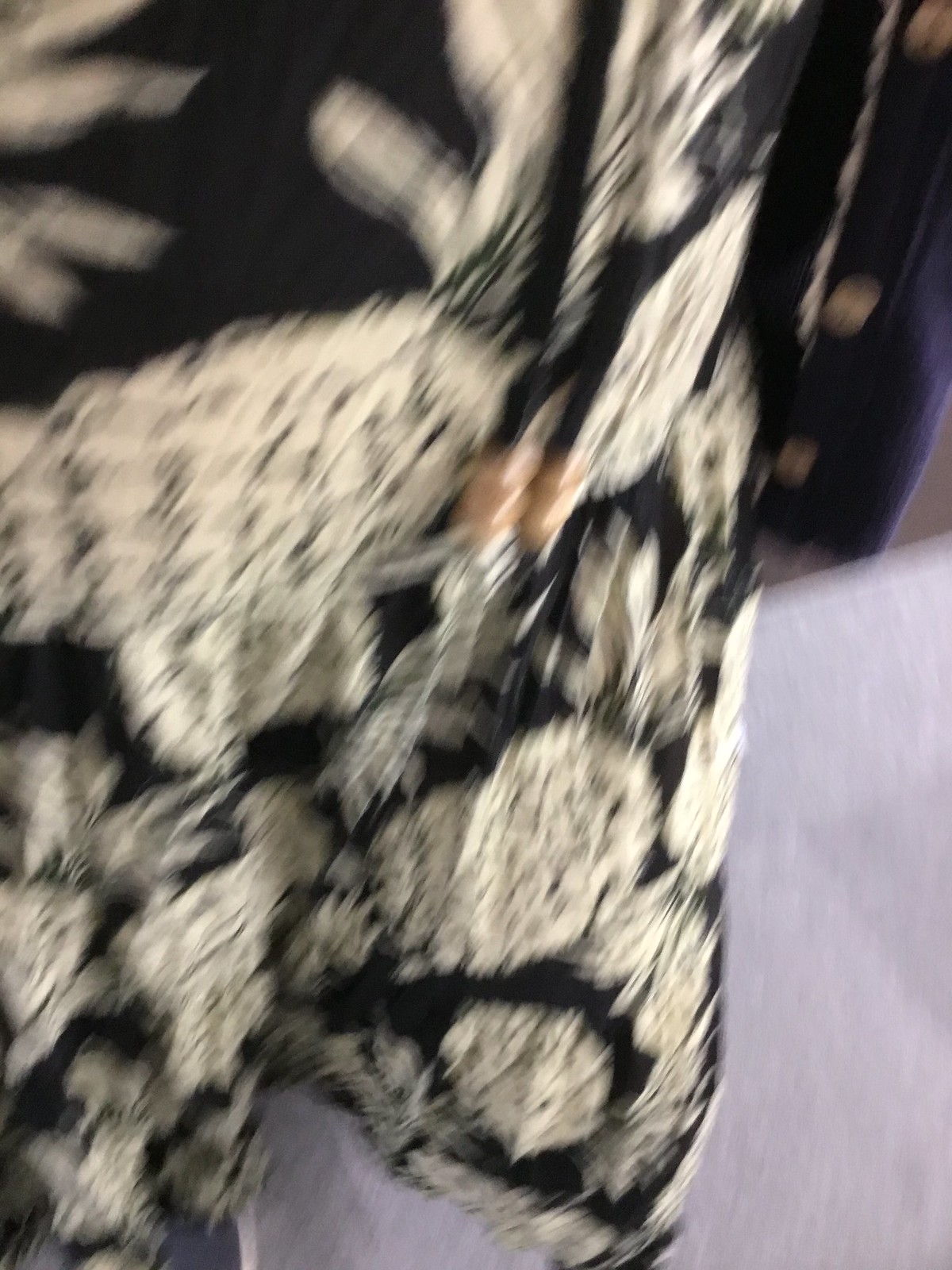This extreme close-up, although very blurry, depicts a black piece of clothing with intricate golden designs that resemble pineapples or floral patterns. There's a visible white surface in the lower right corner with a black object above it, set against a beige or light brown background. On the left side, there’s a portion of black cloth adorned with golden designs, further adding to the garment's pattern. In the middle of the image, there's an indistinct orange or light brown object. The setting includes elements that might suggest a carpeted floor, with hints of a purple piece of furniture and possibly a black dresser in the background. The clothing item, potentially a dress or pants, seems to be held up, suggesting it might be part of a suit with black and white elements.